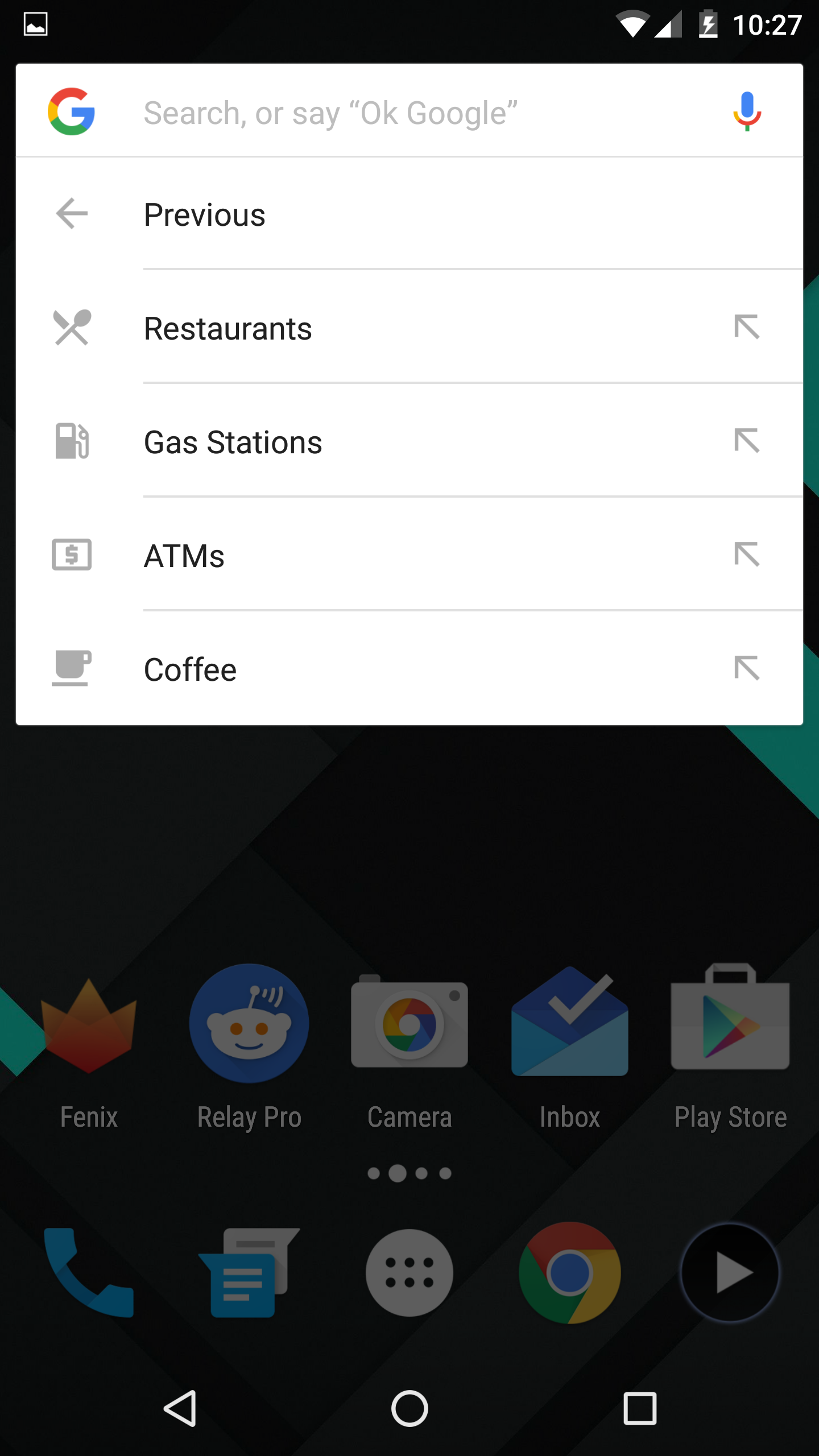A screenshot taken from a cellphone display features a prominent white overlay box at the top, set against a black background. Inside the white box, the recognizable multicolored capital 'G' for Google is prominently displayed at the top left, followed by the grey text, "Search or say 'OK Google'," alongside a microphone icon. Below this search prompt, there is a navigation bar with icons representing various categories: 

- An arrow pointing left, indicating a 'Back' function.
- A crossed spoon and knife with the label "Restaurants."
- A gas pump icon labeled "Gas stations."
- An icon of dollar bills in a box labeled "ATMs."
- A coffee cup icon labeled "Coffee."

On the right side of this bar, there are four small arrows pointing diagonally up towards the left corner, also in grey. The top of the screen displays the time as 10:27, and a battery icon shows that the phone is charging, despite the battery being low. A few additional status icons can be seen at the top. At the bottom of the screen, two faint rows of app icons are partially obscured by the white overlay box.